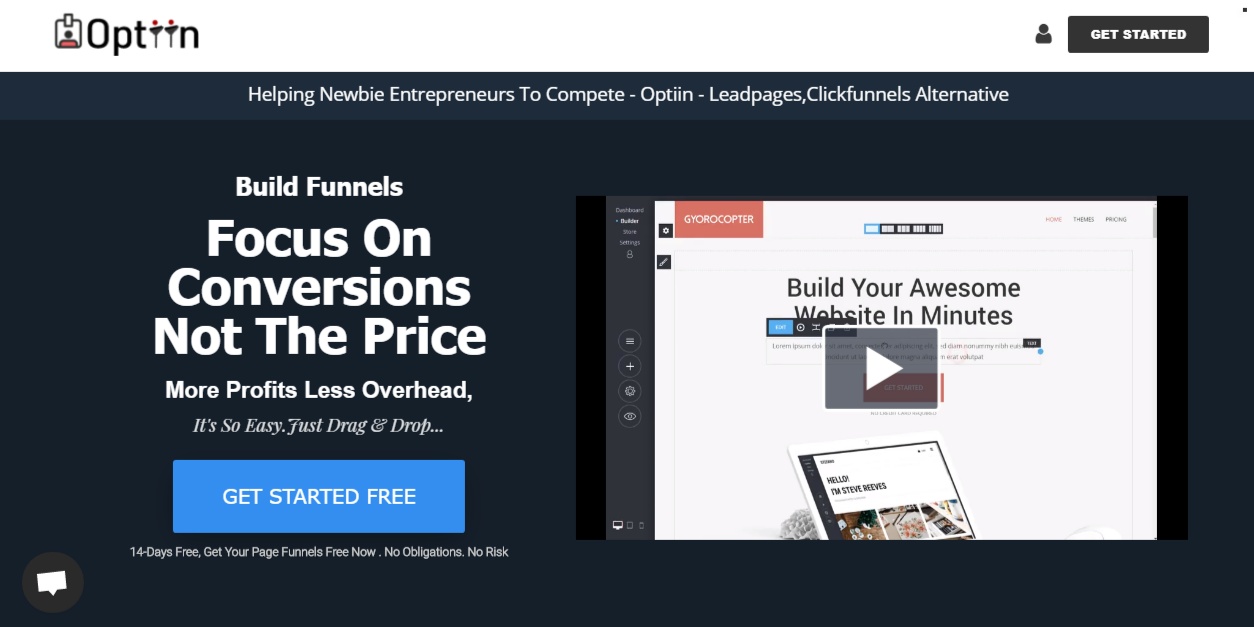This image is a screenshot of a web page dominated by a lot of negative space. At the top left, a small icon and a logo spell out "O-P-T-I-I-N" on a white background. In the upper right corner, against the same white backdrop, is a black button featuring white text that reads "Get Started" alongside a small person icon.

The primary content of the page is set on a dark blue background. On the left side, white text encourages users by stating: "Build funnels. Focus on conversions, not the price. More profits, less overhead. It's so easy, just drag and drop." Below this text is a vibrant blue button that reads "Get Started Free", accompanied by a smaller note in white text below it that promises "14 days free. Get your page funnels free now. No obligation. No risk."

On the right side of the dark blue area, there's a video screenshot marked by a play button in the center. The video promotes the simplicity of creating a website, suggesting users can "build your awesome website in minutes."